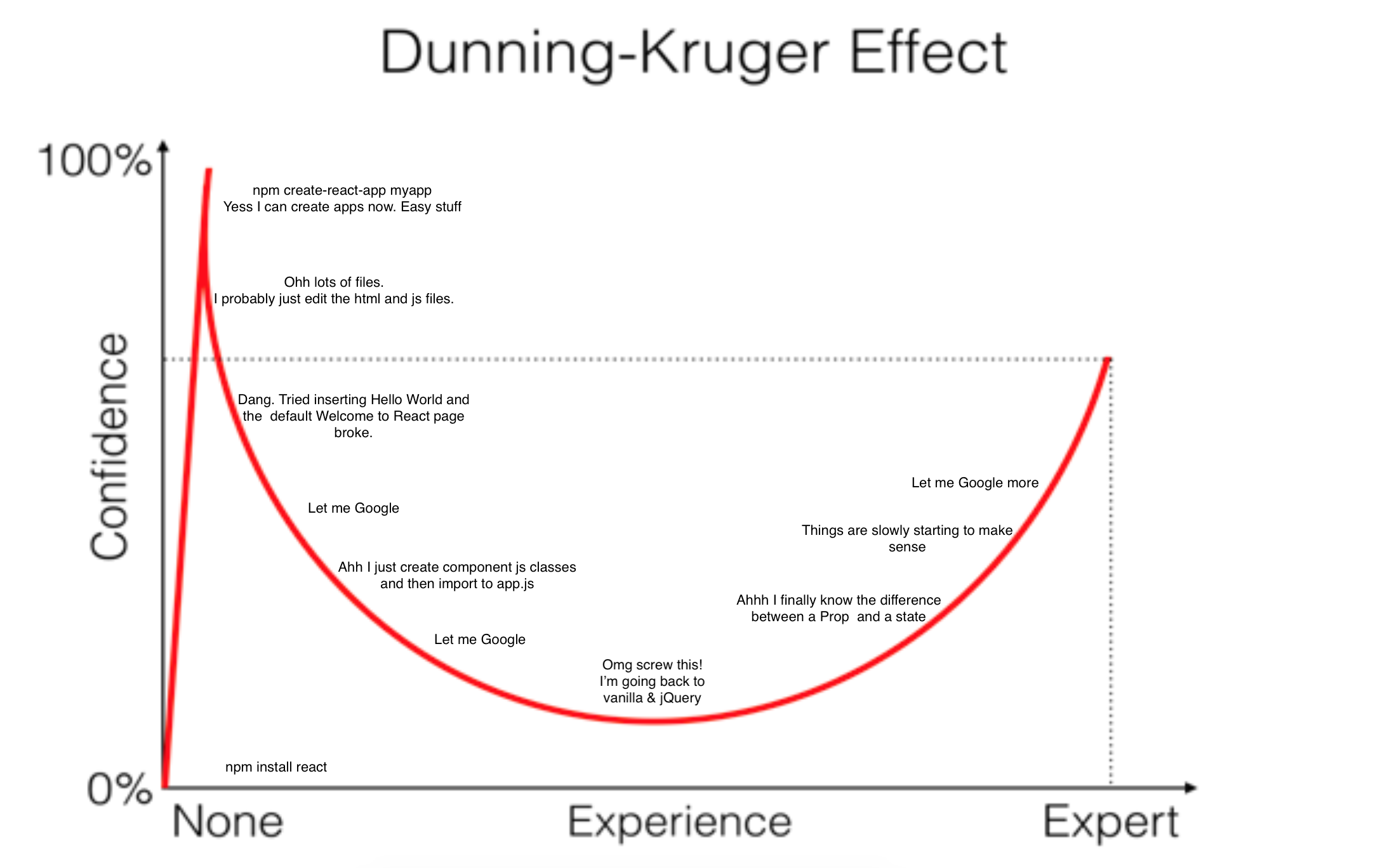The image is a vertically oriented infographic with a plain white background, likely displaying on a computer screen. At the top, in black letters with only the initial letters capitalized, it reads "Dunning-Kruger Effect." Below this title, a chart is shown featuring two axes: a horizontal one labeled "Experience" and a vertical one labeled "Confidence," each with respective arrows indicating direction.

The horizontal axis of the chart has "0%" on the far left (indicating no experience) and "100%" on the far right (indicating expert-level experience). The vertical axis starts with "0%" at the bottom (indicating no confidence) and reaches "100%" at the top (indicating full confidence). 

Spanning these axes is a red curve that initially rises steeply, peaks early, then descends and gradually levels off into a more gradual upward climb, resembling a semicircle or bell curve. Annotated along this curve are various phrases illustrating different stages of understanding and behavior, including "Let me Google more," "Things are slowly starting to make sense," "O, lots of files," and "I probably just edit the HTML and JS files." These annotations, positioned around the curve, illustrate typical thoughts and actions experienced along the path of gaining expertise within the context of the Dunning-Kruger Effect.